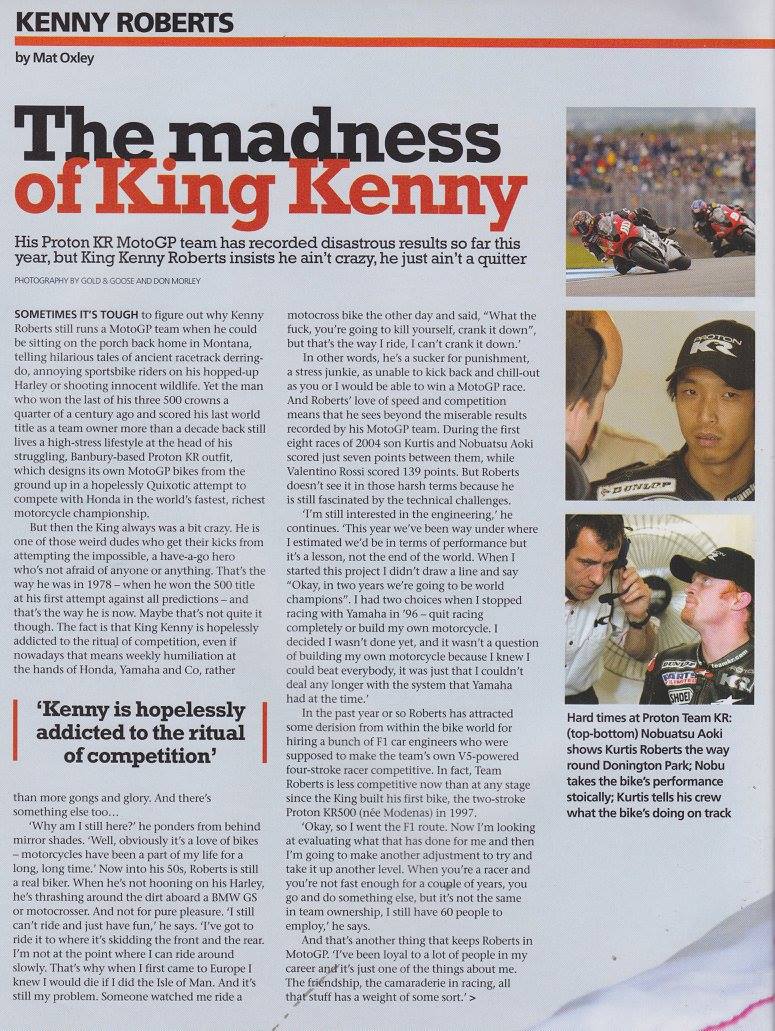The page from the magazine features a light blue, hazy sky background contrasting with a bold headline. At the top left, in prominent black letters, it reads "Kenny Roberts," followed by a thick red line stretching across the width of the page. Beneath the line, in smaller black letters, the byline credits the article to Matt Oxley. The main title, "The Madness of King Kenny," is strikingly divided with black and red text, emphasizing the dramatic nature of the story. 

Below this headline, a brief summary states, "His Proton KR Moto GP team has recorded disastrous results so far this year, but King Kenny Roberts insists he ain't crazy, he just ain't a quitter." A notable quote embedded within the text highlights, "Kenny is hopelessly addicted to the ritual of competition." 

The article is divided into two columns of text, detailing the trials and tribulations of Kenny Roberts and his team. On the right side of the page, there are three square photos. The first depicts two motorcycles leaning sharply into a turn during a race. The second image shows a young man wearing a black hat, and the third features a fair-skinned man with a red beard next to another individual in a white shirt with a headset. The caption for these images reads, "Hard times at Proton Team KR. Top to bottom: Nobuatsu Aoki shows Curtis Roberts the way around Donington Park. Nobu takes his bike's performance stoically. Curtis tells his crew what the bike's doing on track." The visuals and text together paint a vivid picture of the struggles and steadfast determination within Kenny Roberts' racing team.